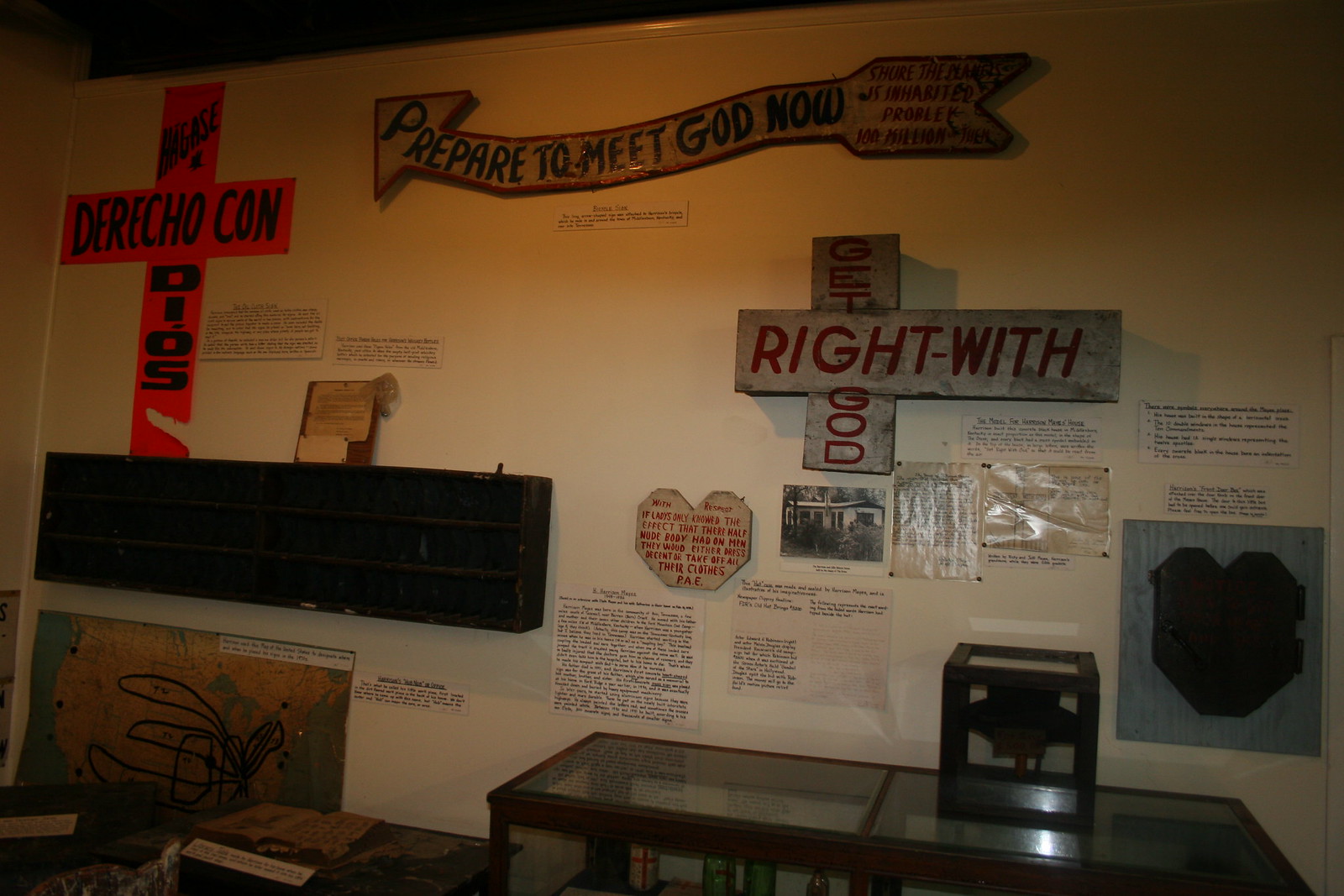The photograph depicts the dimly lit interior of what appears to be a religious exhibit, possibly set up in a museum or church. The space is illuminated primarily by a single overhead light, casting a subtle glow over the scene. Dominating the backdrop, a white wall is adorned with various small squares of paper, featuring text and images that are too small to decipher clearly. Among these, two heart-shaped posters stand out with unreadable inscriptions.

In front of this wall, a glass display case, framed in brown, takes center stage. Atop this case sits another smaller glass case. Prominently featured in the exhibit are several religious-themed items, including a red cross made out of paper bearing an unreadable message in a foreign language. Adjacent to it, a wooden sign nailed to a board, displays the message "Get right with God," and above it, a wooden cut-out arrow directs viewers to "Prepare to meet God now" in black letters. Multiple art pieces and white signs with unreadable black text complement the display, contributing to the contemplative atmosphere of the exhibit.